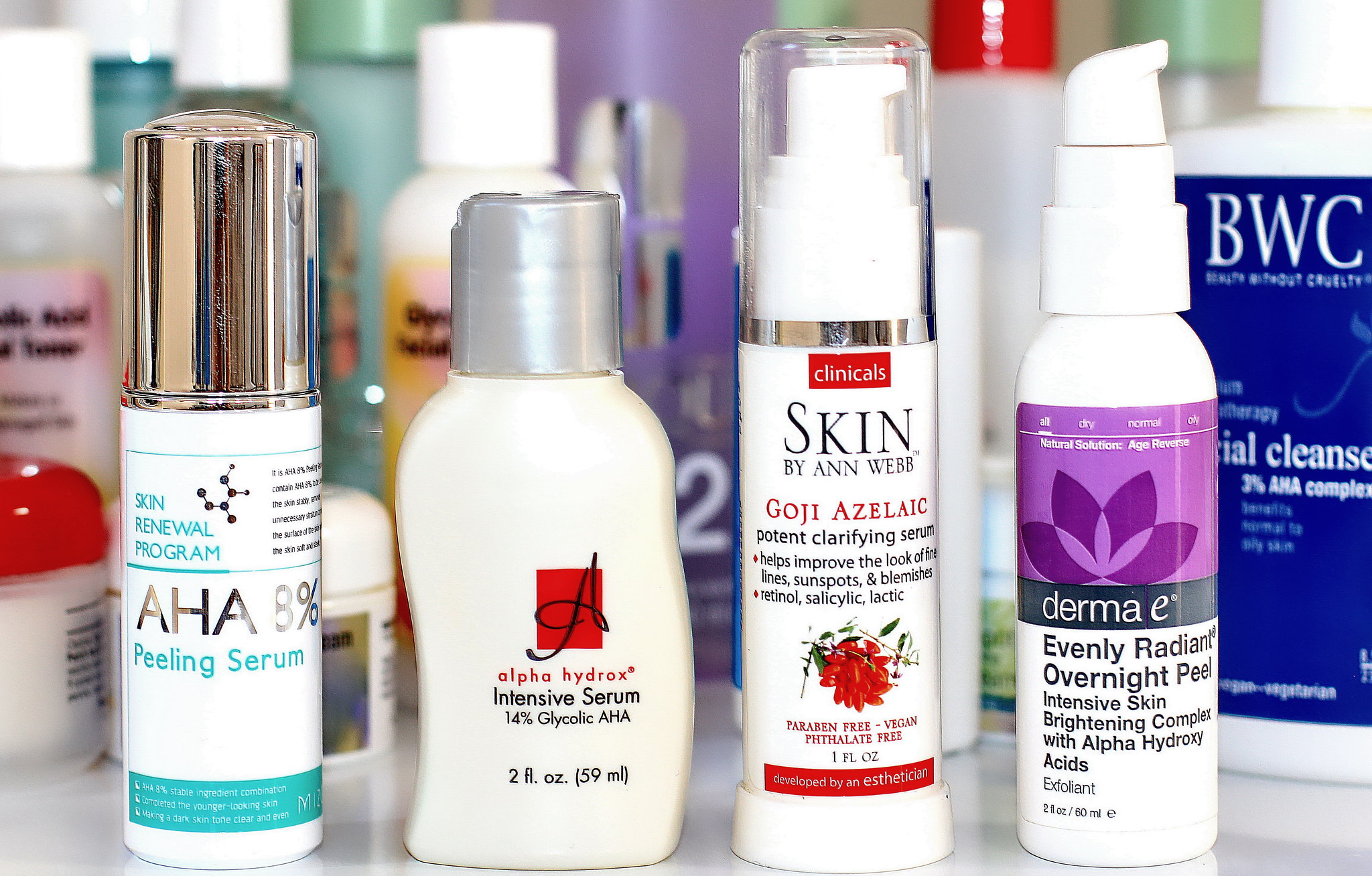This image is a detailed photograph showcasing an array of skincare products on display in a retail setting. Among the items, there are two jars positioned in the bottom left-hand corner. The first jar contains a white substance and features a red lid, while the adjacent jar is also white but has a matching white lid. 

The rest of the display consists of several plastic bottles, some with screw-on white lids and others with pump dispensers. Notably, the bottle on the far right has a white pump dispenser, while the second bottle to the right also has a pump dispenser covered by a clear cap. 

From the top left, there are fourteen bottles, each with distinct labels. The four bottles in the front row have the following descriptions:

1. The first bottle is labeled "Skin Renewal Program AHA 8% Peeling Serum."
2. The second bottle reads "Alpha-Hydrox Intensive Serum 14% Glycolic AHA, 2 fluid ounces (59 milliliters)."
3. The third bottle is branded "Clinical Skin by Ann Webb Goji Azelaic," describing it as a potent clarifying serum that helps improve the appearance of lines, sunspots, and blemishes containing retinol, salicylic acid, and lactic acid. It is paraben-free, vegan, and phthalate-free, with a volume of one fluid ounce. It is noted to be "Developed by an esthetician."
4. The fourth bottle is labeled "Natural Solutions Age-Reverse Derma E Evenly Radiant Overnight Peel," an intensive skin brightening complex with alpha hydroxy acids as an exfoliant, provided in a two fluid ounce (60 milliliters) bottle.

In the background to the right, the word "Cleanse" is visible, indicating this section may house cleansing products.

The detailed arrangement and variety of products suggest an extensive selection catered to different skincare needs, possibly in a dedicated skincare retail environment.